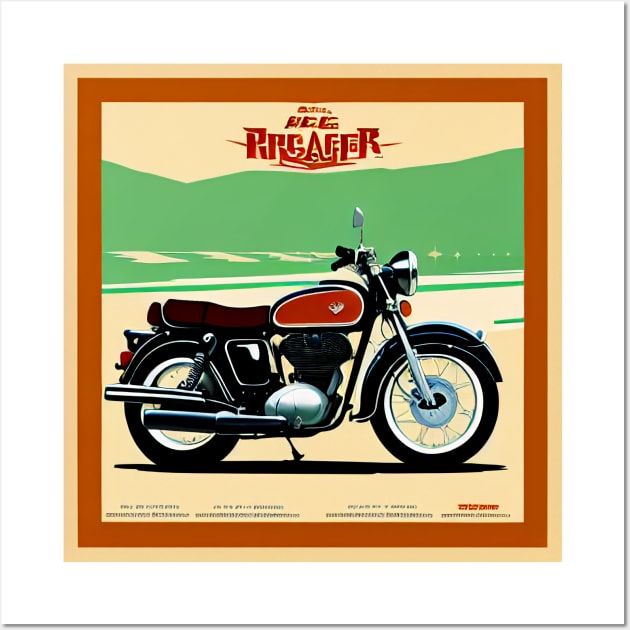This digitally illustrated album cover features a sleek, modern motorcycle prominently displayed against a tan background. The motorcycle, characterized by its black tires, shiny gray headlight, marine-colored seat, and red gas tank, appears almost new. Encircling the artwork is a double brown frame, with a lighter outer section and a darker inner section, providing a subtle but distinct border to the composition. The motorcycle, rendered to face the right, stands against a backdrop that suggests abstract green hills or perhaps the green hue of coastal water, adding an impressionistic and somewhat ambiguous element to the scene. At the top of the image, red text begins with what appears to be an "R," but the unique, chunky font makes it nearly impossible to decipher, as the letters bleed together into an unreadable smear. Similarly, at the bottom of the image, small text is present but remains indistinguishable and nonsensical, providing no clear message. This generative AI creation combines vivid colors and abstract elements, offering a visually intriguing but cryptic presentation reminiscent of an album cover.